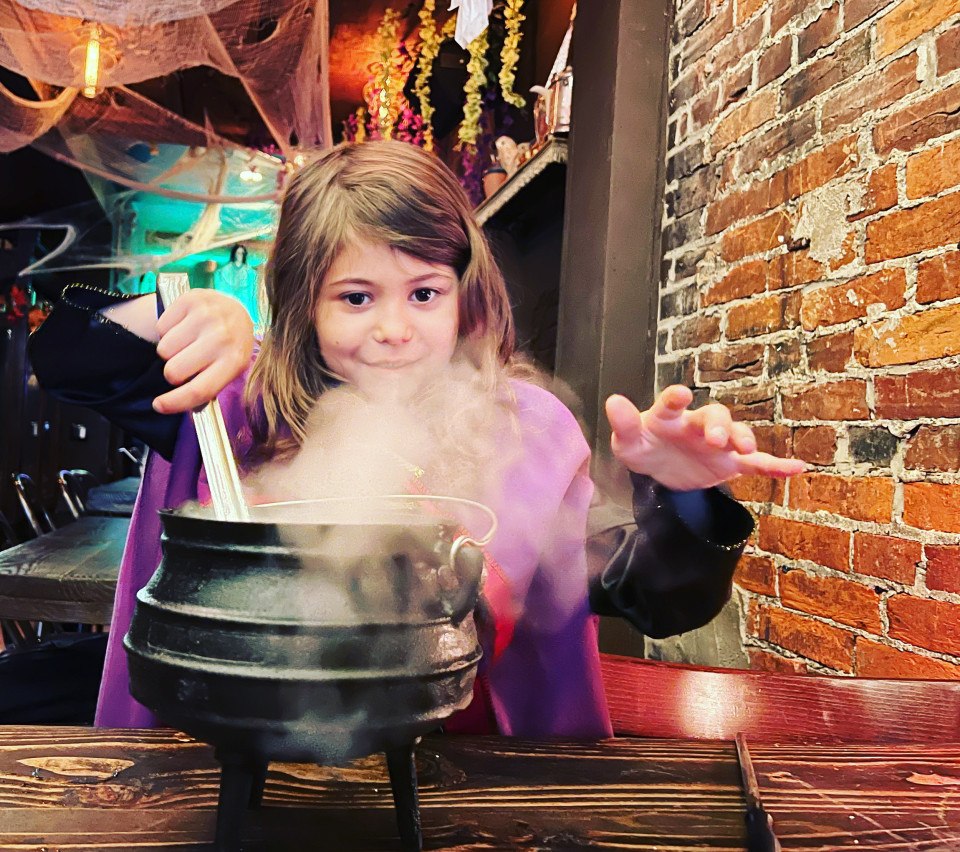The image depicts a joyful little girl, likely between the ages of six and eight, with shoulder-length hair that is a mix of brown and blonde. She has dark eyes and a round face, with a wide, mischievous smile as she looks at the camera. She is dressed in a purple cape with black sleeves, reminiscent of a witch's costume, which suggests she is participating in a Halloween activity or event. 

In front of the girl is a wooden table on which sits a small black cauldron. She is holding a silver ladle or spoon with both hands, stirring the cauldron from which steam or smoke is rising. 

To her side is an old, exposed red brick wall with some kind of dark brown metal piece attached to it. The background is adorned with Halloween decorations, including fake spiderwebs draped across the ceiling. There is a hint of turquoise and some green leaves and pink flowers hanging behind her, suggesting a festive atmosphere. The scene captures the whimsical essence of Halloween, with the little girl reveling in her role as a young witch brewing a magical potion.